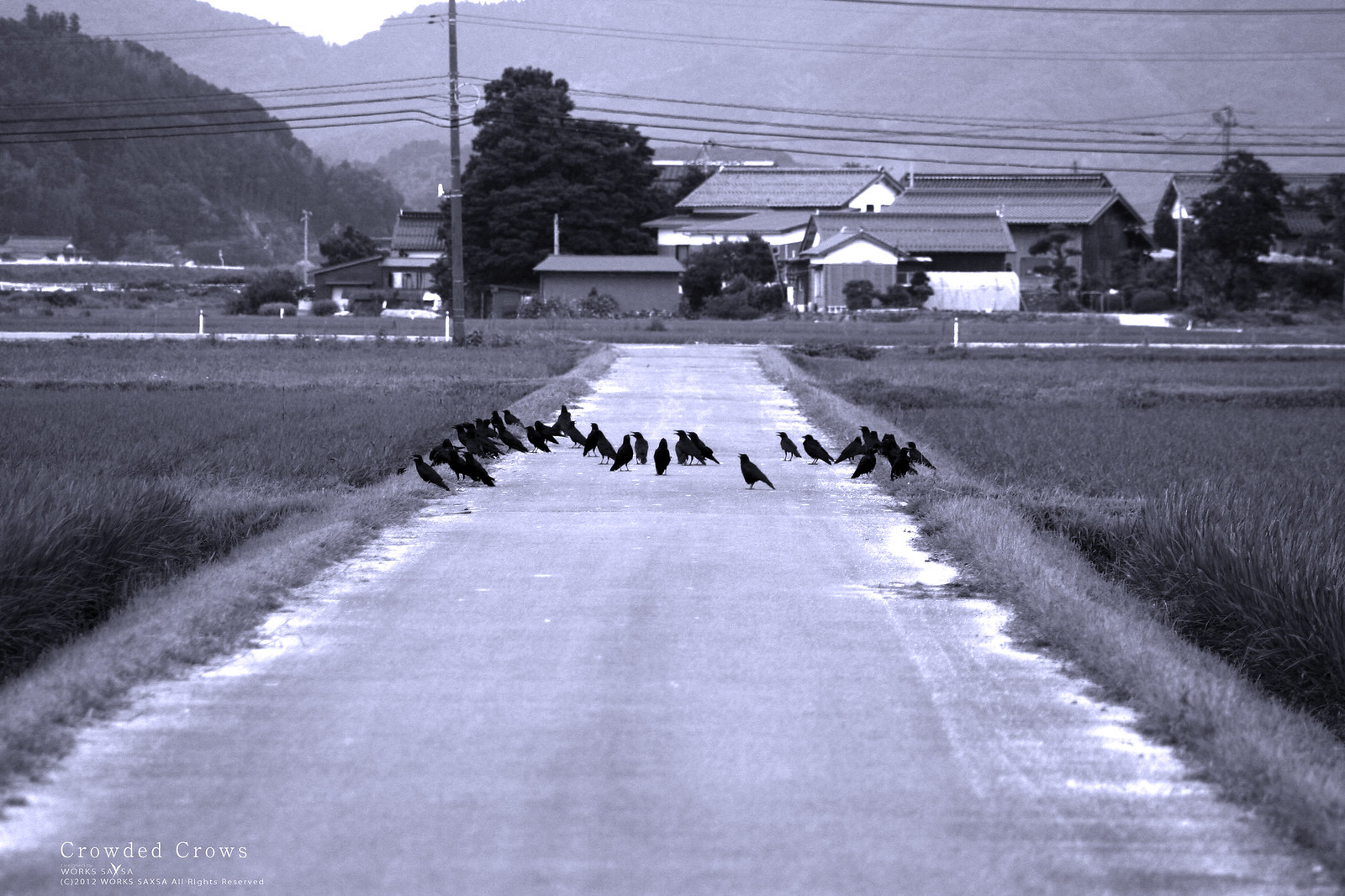This black-and-white photograph, titled "Crowded Crows," captures a serene countryside road scene dominated by nature and a peculiar congregation of birds. The narrow road stretches through tall grass flanked by bushy patches on both sides, devoid of any cars or people. In the center of the road, approximately 25 blackbirds, likely crows or a similar species, are aligned together, appearing to cross from right to left. Behind them, quaint one- and two-story farm buildings with pointy roofs cluster on the left side, accompanied by a large, lush tree and telephone poles with wires crisscrossing above. The background is graced by imposing, tree-and-grass-covered hills, enhancing the rural ambiance. A watermark in the bottom left-hand corner reads "Crowded Crows," followed by "Works S-A-X-S-A © 2012 All Rights Reserved."